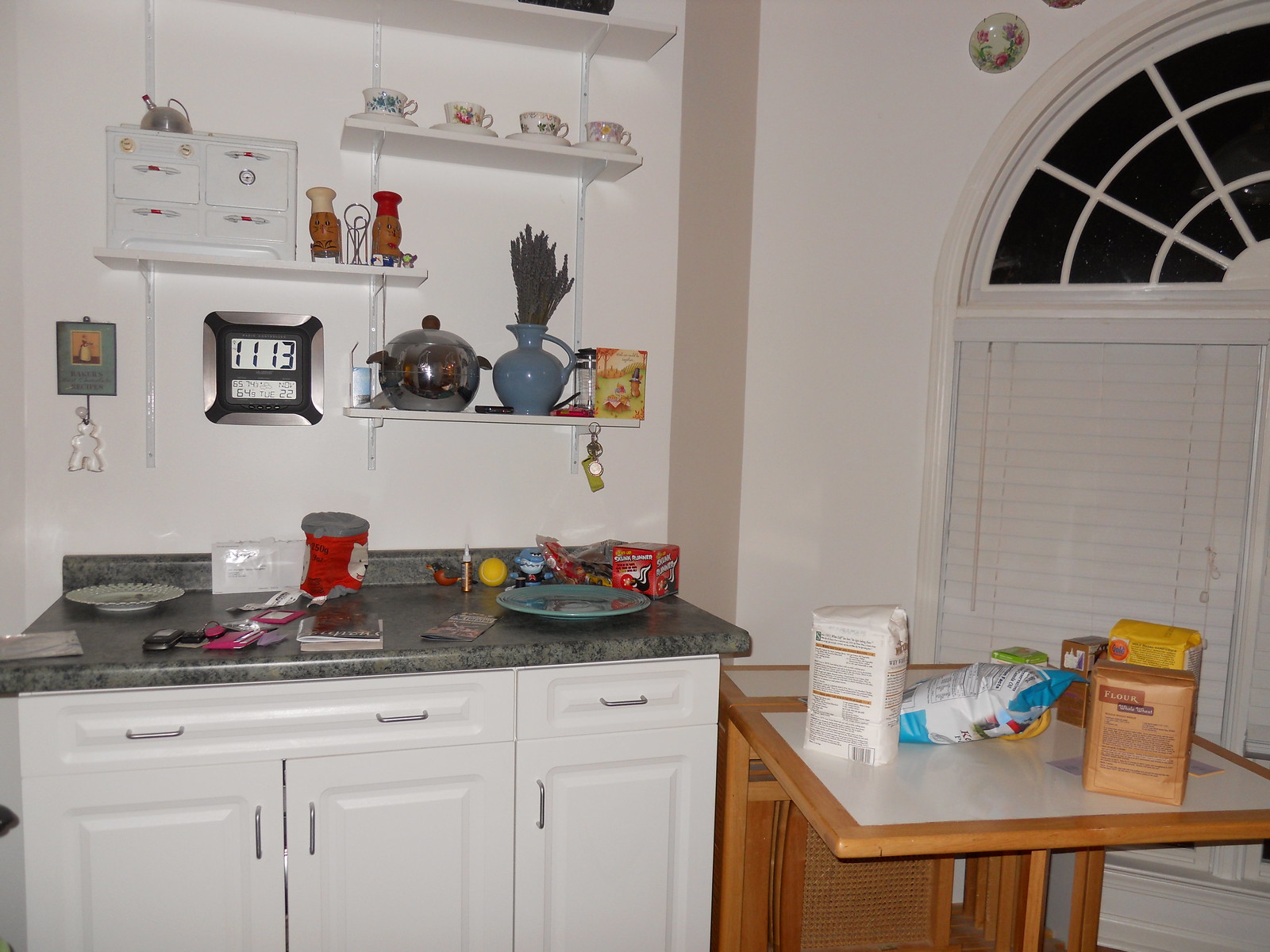A bustling kitchen filled with various gadgets and ingredients. On the left-hand side of the image, three metal struts support an array of shelves at differing heights. The middle shelf features a charming, decorative faux oven in white, adorned with a miniature tea kettle. Beside this oven sit whimsical salt and pepper shakers, fashioned to resemble brown eggs. Above, a higher shelf holds four colorful teacups: some showcase white porcelain with blue imprints, while others display bright orange and sunny yellow patterns.

Below these two shelves, a lower one hosts a silver pot with sturdy black handles. Adjacent to the pot, a blue vase with an ornate handle and a bulbous base tapers elegantly, housing a sprig of sage or mint. A box of crackers, likely Triscuits, rests nearby.

The countertop beneath is a striking green and black marble-like surface, though seemingly crafted from faux materials. Underneath, a white cabinet with three doors and two drawers holds various kitchen essentials. The left drawer is noticeably larger than the right. Atop this cabinet lie a cluttered assortment of plates, coffee canisters, ingredients, a cell phone, and keys – essentially a catch-all for daily necessities.

To the right of the cabinet, a brown table with a tan top is crowded with baking supplies. A bag of flour, various types of cake flour, crackers, and chips are strewn across, poised for culinary use. The scene exudes a warm, lived-in atmosphere, indicative of frequent and enthusiastic cooking.